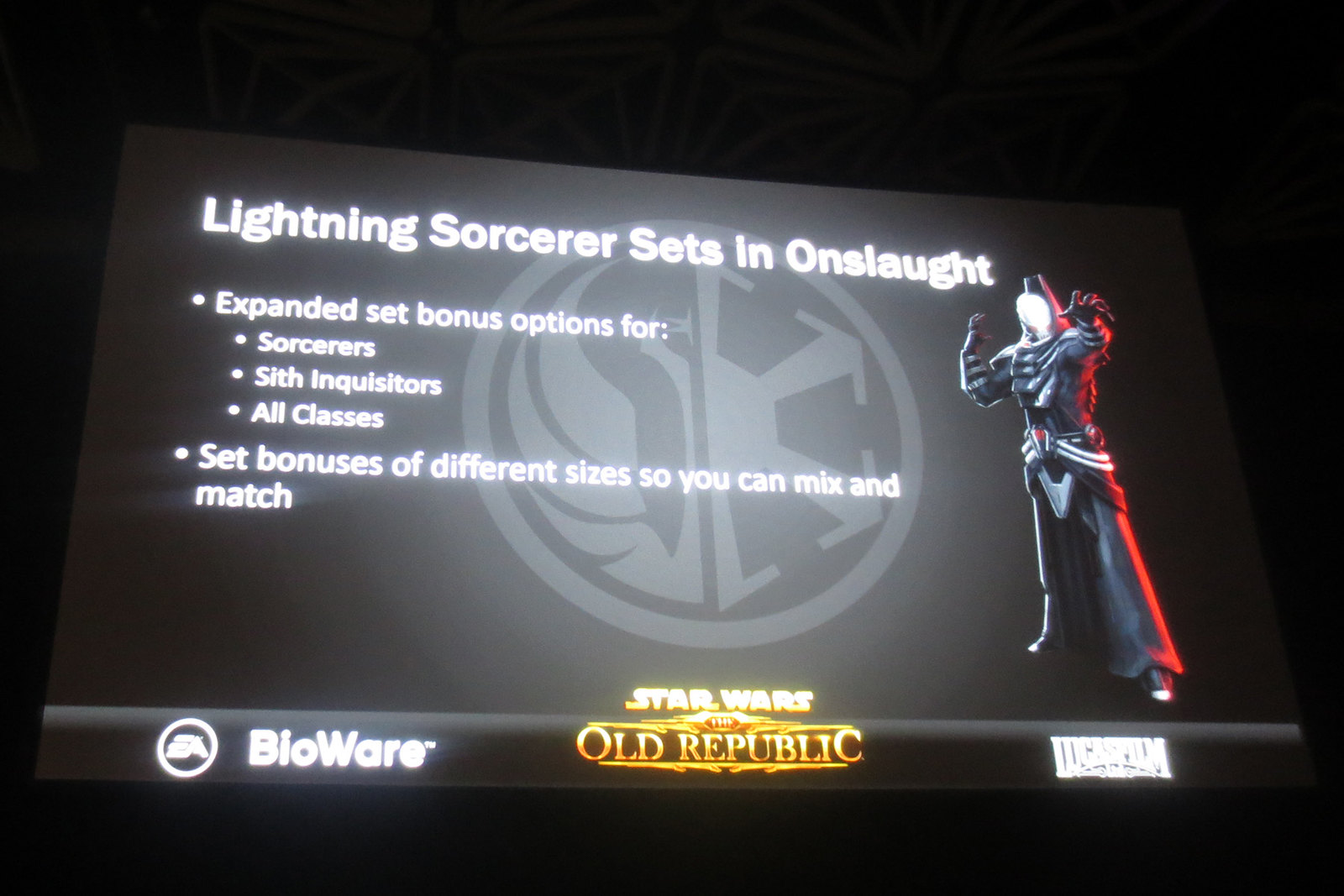The image is a computer-generated graphic, likely a screen capture from a video game reminiscent of a website or digital interface. The primary color scheme of the image is black and gray, with a black background and gray inserts. Prominently, the text "Lightning Sorcerer Sets in Onslaught" is displayed in white at the top, followed by "Expanded Set Bonus Options for Sorcerers, Sith Inquisitors, All Classes" and "Set Bonuses of Different Sizes so you can Mix and Match." The centerpiece graphic features a faceless character dressed in red and black, likely representing a Sith warrior. A logo resembling a dragon or bird of prey appears nearby. At the bottom of the image, three logos are aligned: the BioWare logo to the left, the Star Wars: The Old Republic logo in the middle, and the Lucasfilm logo to the right. The overall impression is of a promotion or informational graphic related to a video game, specifically within the Star Wars universe.